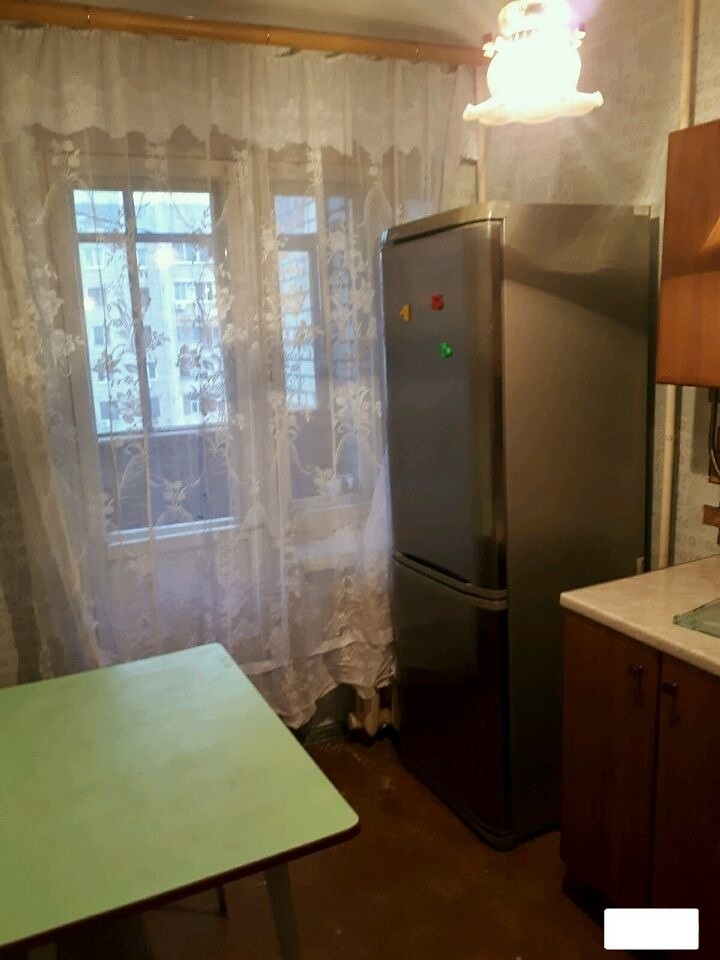This color photograph captures the corner of a small kitchen. Dominating the scene is a stainless steel refrigerator adorned with colorful letter magnets, situated next to brown wooden cabinets with a white countertop, likely quartz. In front of the cabinets stands a simple green table with a possible Formica surface. The kitchen features brown wooden floors and a light fixture above, characterized by a white tulip-shaped globe. The window in the background, dressed in lace curtains on a large wooden rod, reveals a view of another building outside. Hints of a radiator are tucked away in the corner behind the refrigerator, partially obscured by the curtains.